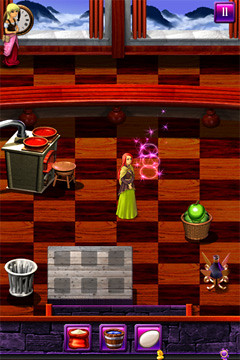The detailed image displays a vibrant and highly saturated pixel art screenshot from a video game. Dominating the screen is a colorful interface that invites players into a lively world. In the upper right corner, a hot pink and purple square with white vertical lines serves as the pause button. The top of the screen showcases windows that frame a picturesque snowy mountain landscape and fluffy clouds, enhancing the whimsical ambiance.

In the upper left, a character icon featuring a blonde person who appears to be a girl stands against a clock backdrop, possibly indicating a timer. The checkerboard floor at the bottom provides a stage for various colorful elements. Prominently featured in the center is a woman with red hair, draped in a light brown shawl over a dark purple top and a flowing green dress. Behind her hovers a translucent bubble.

On the left side of the image, a gray stove with two cauldrons containing red liquids is seen, accompanied by a stool in front of it. A silver bucket and a round brown bucket filled with a green substance are also visible. To the right, a basket brimming with green apples rests on the floor. The lower left corner of the screen has a wastebasket, while the bottom of the screen displays several icons representing game elements, including a flower, an egg, and a bucket.